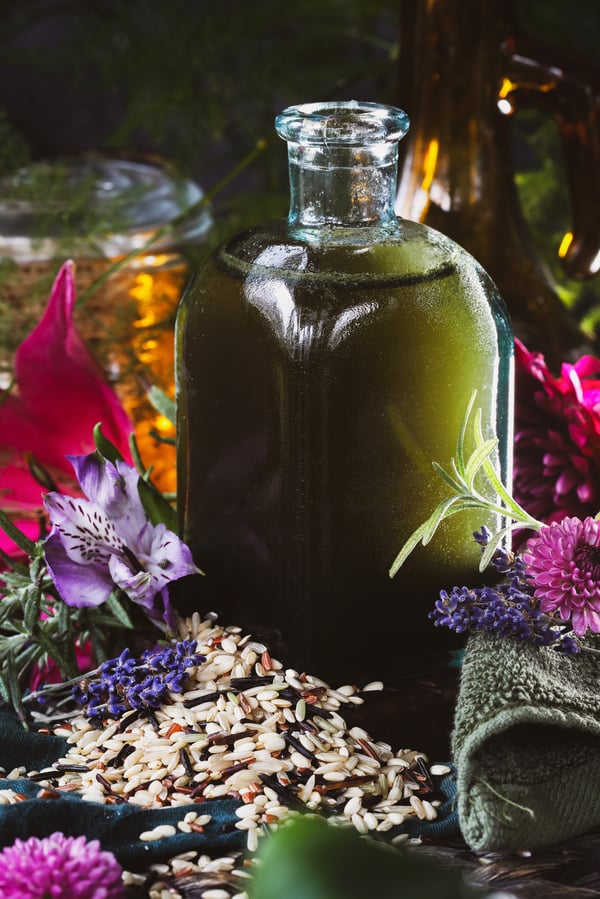This close-up, aesthetically pleasing photograph centers on a clear glass bottle with a thick body and a narrow neck, containing a dark, cloudy green liquid. Surrounding the bottle are various decorative elements: a small purple iris flower to the front-left, tiny grains of white and black rice at its base, and different shapes and colors of seeds. To the right of the bottle, a green terry cloth towel is neatly folded, adorned with a pink flower, a purple flower, and a small sprig of grass. The background is blurred but hints at additional glass containers with various colored liquids, adding depth and intrigue to the scene. The vibrant palette and carefully arranged objects suggest the photograph could be part of a product or food shoot, emphasizing its decorative and visually striking nature.